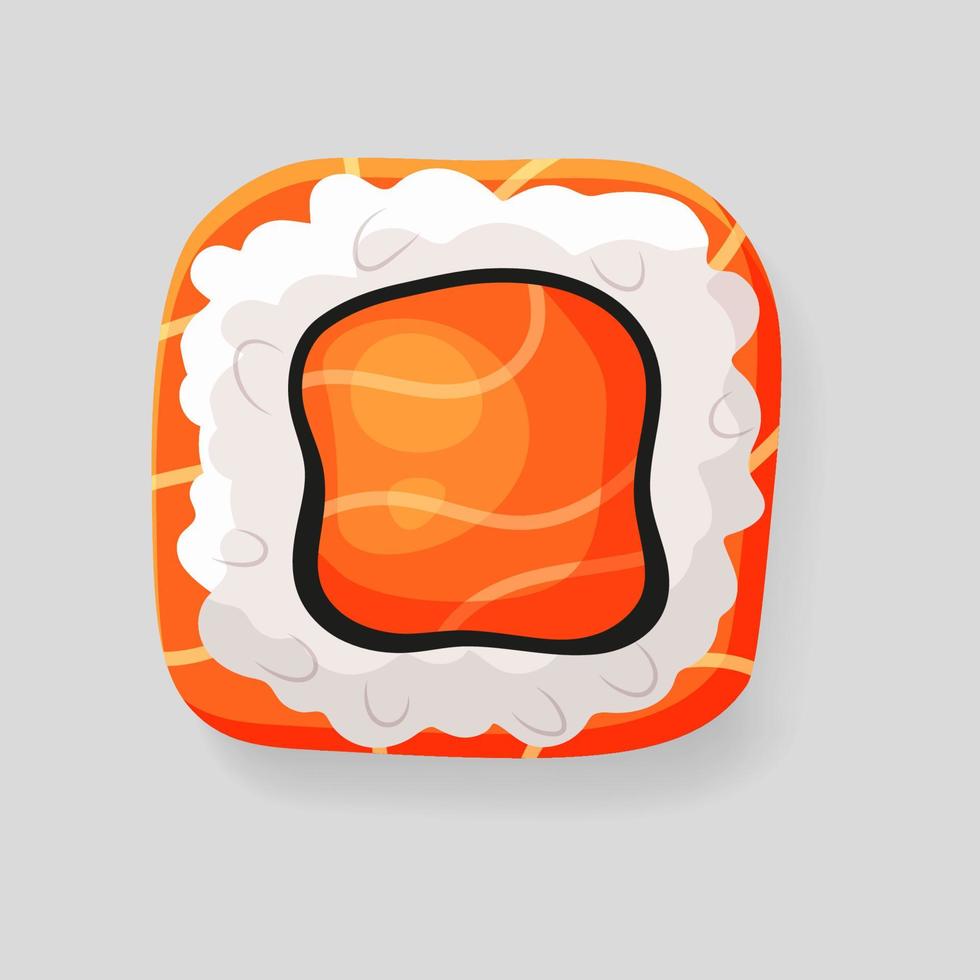The image features a computer-generated graphic set against a gray background. Central to the composition is an abstract, square shape with curved corners, predominantly colored in varying shades of orange. The right side of the square transitions into a dark orange hue while the left side presents a lighter orange shade, both wrapped in a pattern of yellow stripes that add complexity and texture. 

Overlaying this design is what appears to be a fluffy, white cloud-like form, reminiscent of whipped cream. Additionally, the white area contains black and orange elements, including squiggly lines and small circular shapes, which together evoke the appearance of an animal cell or possibly a dessert. The image, abstract in nature, could also be interpreted as a whimsical piece of toast or candy, emphasizing its versatility and imaginative quality.